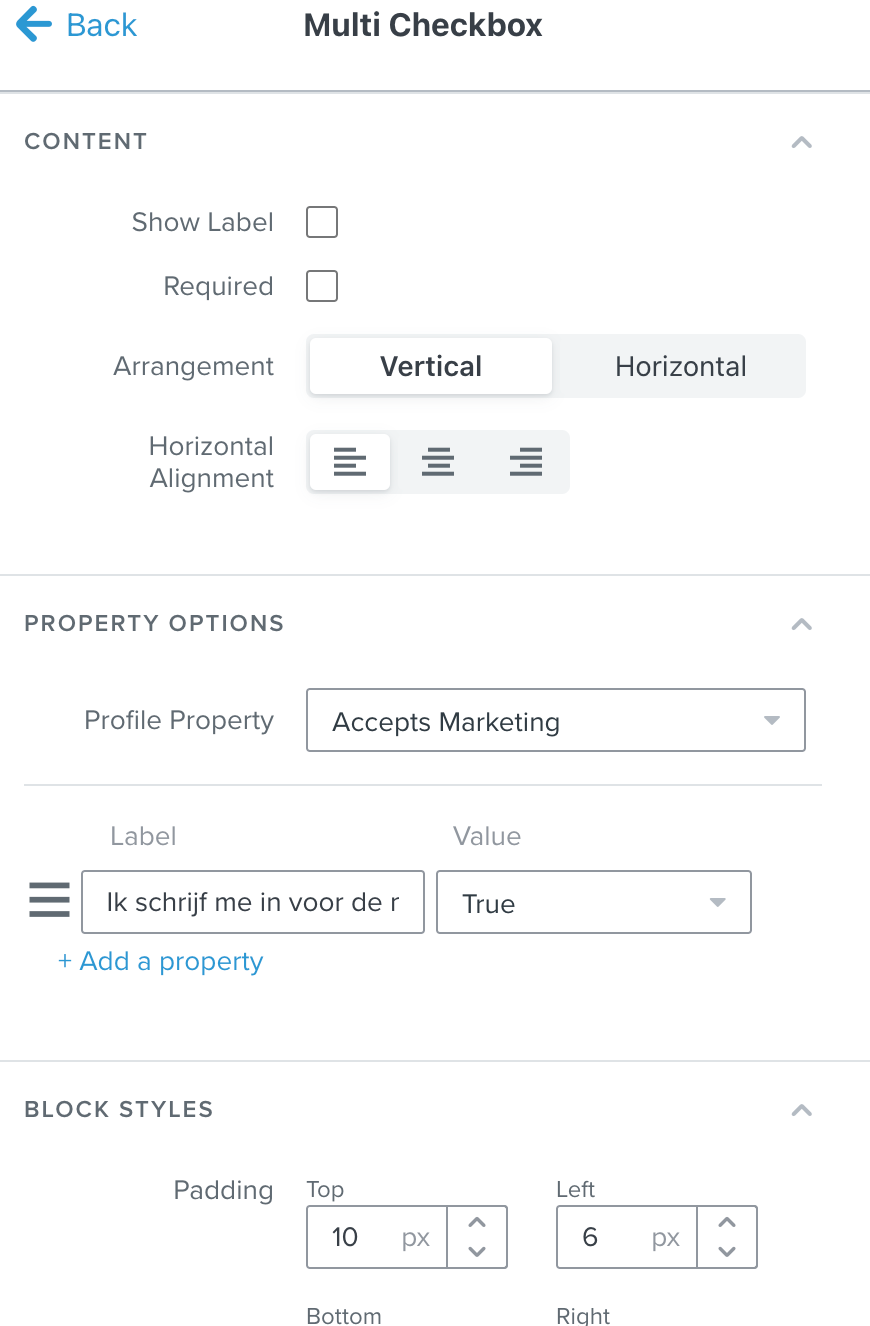Set against a white background, this screenshot captures the upper left corner of a software interface. In the top-left corner, a blue "Back" button with a left-pointing arrow is visible. To its right, centered, is the bold black text "Multi Checkbox." Below this, a light gray horizontal line divides the section.

Underneath the line, there are options related to "Content." The options "Show Label" and "Required" are present, each accompanied by a small gray checkbox. 

Next to "Arrangement" on the right, the options are listed as "Vertical" and "Horizontal," with additional layout alignment choices to the right. Another gray horizontal line further divides the section.

Below this line, the "Property Options" section is highlighted, with fields like "Profile Property" and an "Action Button" labeled "Accepts Marketing" that features a dropdown menu.

Beneath this, there are two input boxes side-by-side, labeled "Label" on the left and "Value" on the right. At the bottom of the image, the term "Block Styles" is indicated, followed by the parameter "Padding."